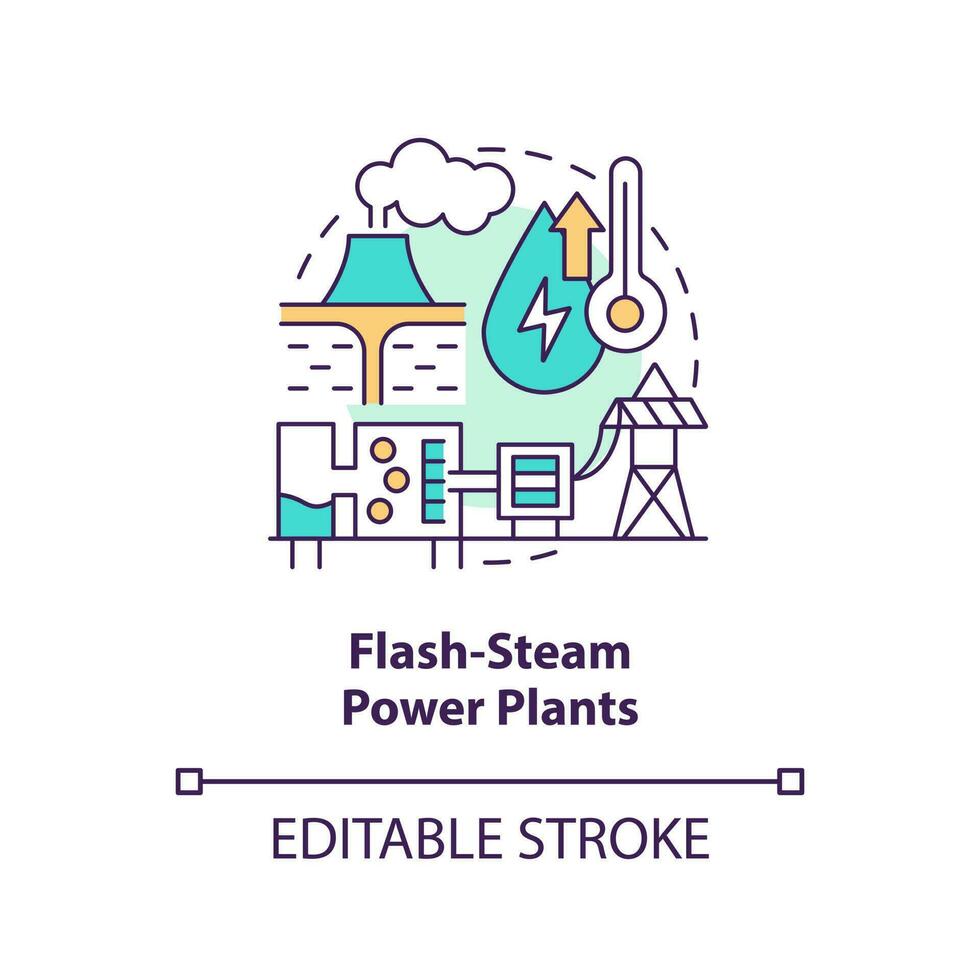This is a detailed, hand-drawn diagram depicting the inner workings of flash steam power plants. The illustration is more cartoonish than to scale, featuring several interconnected elements. At the top, a blue-green cooling tower emits steam into the air, depicted as a cloud intersected by dashed lines that connect to a yellow thermometer and a rising arrow symbolizing temperature increase. The backdrop is a tannish-orange hue.

Central to the diagram are a steam generator and a turbine, both integral to the power generation process. The generator features three yellow dots and several blue lines that extend from it, leading to another square structure symbolizing a building. This building, located beneath the smokestack, includes gold dots and connects via dashed lines to the cooling tower, illustrating how steam is converted to electricity.

To the right, a blue droplet with a lightning bolt emphasizes the involvement of water and electricity. The entire setup is interconnected, showcasing the flow from heating water to generating power. Below the visual elements are explanatory texts: "Flash Steam Power Plants" in black letters, with an editable stroke feature highlighted beneath. This informative and visually engaging diagram effectively portrays the mechanics of flash steam power plants.